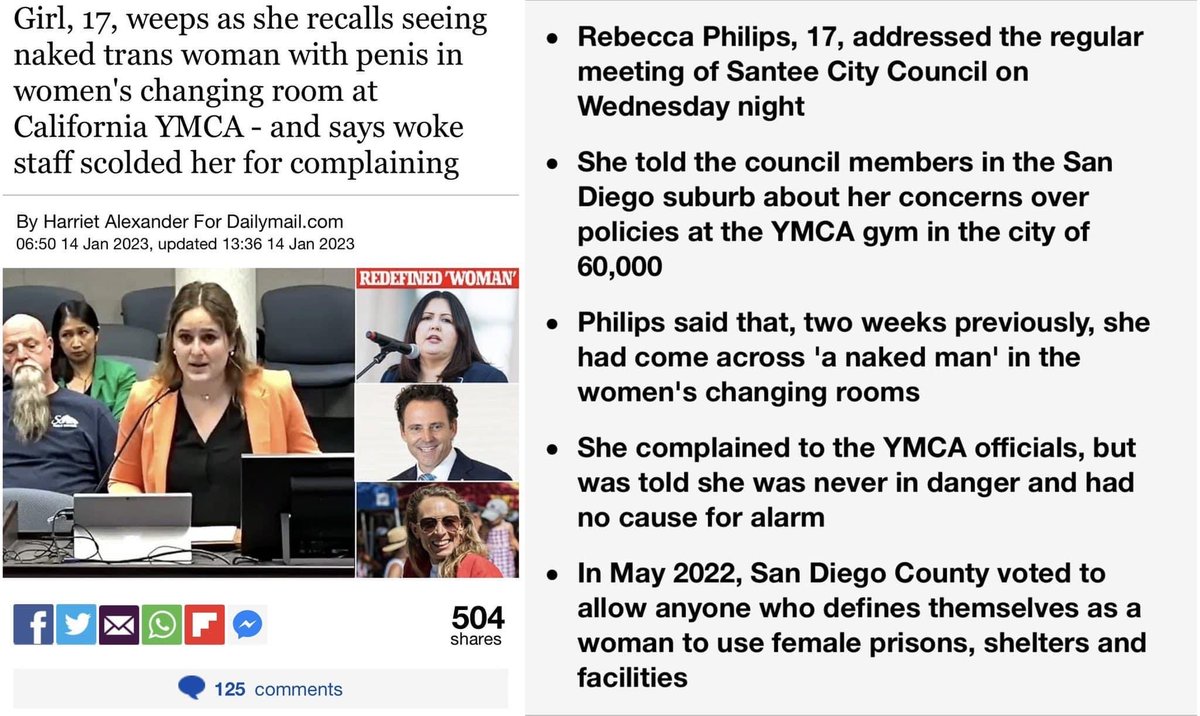This is a detailed and descriptive caption of the image:

---

This screenshot is taken from an unspecified web page featuring a headline: "Girl, 17, weeps as she recalls seeing naked trans woman with penis in women's changing room at California YMCA. Woke staff scolded her for complaining. By Harriet Alexander for DailyMail.com, 6:50 PM, 14 January 2023, updated 1:36 PM, 14 January 2023." 

The central photograph captures a young woman with long brown hair, dressed in an orange blazer over a black top. She appears to be delivering a testimony in a courtroom setting. Seated behind her are individuals including an older bald man with a long gray beard and an Asian woman with long black hair who is looking to her left.

On the right side of the image, there are three smaller images: one showing a woman with long dark hair speaking into a microphone, another of a man looking at the camera with a smile, and a third image of a person with long wavy blonde hair wearing aviator sunglasses and looking at the camera.

Below the main image, it indicates that the content has "504 shares" and "125 comments."

Additionally, text on the right states: "Rebecca Phillips, 17, addressed the regular meeting of Santee City Council on Wednesday night. She shared with the council members in the San Diego suburb about her concerns regarding the policies at the YMCA gym in the city of 60,000. Phillips recounted that two weeks prior, she encountered a naked man in the women's changing rooms. When she reported this to YMCA officials, she was informed that she was never in danger and had no reason for alarm. In May 2022, San Diego County voted to permit anyone identifying as a woman to access female prisons, shelters, and facilities."